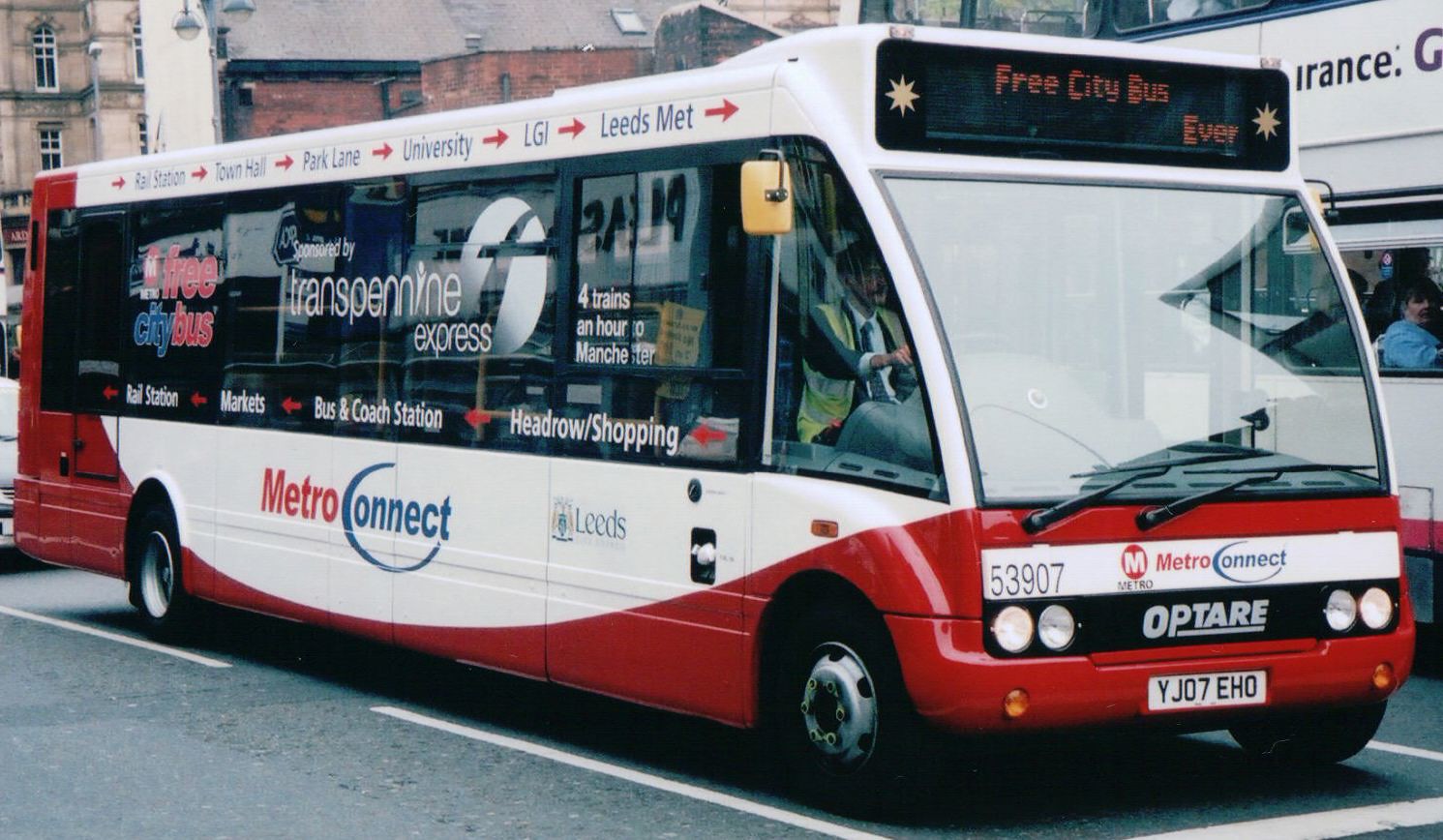This detailed photograph features a red and white bus, prominently displaying the name "MetroConnect" on its front and sides. Positioned in the midst of traffic, the bus's front facade includes a big square window, below which the grill is labeled "Optair." Just above the grill, a white strip clearly states "MetroConnect." On the side panel, vibrant advertisements for TransPennine Express can be seen, along with repeated mentions that it is a "Free City Bus." A sticker on the back window reaffirms this, while an LED display at the front top also highlights the "Free City Bus" service. The bus route includes stops from the rail station to the Town Hall, Park Lane, University, LGI, and Leeds, aimed at facilitating easy transit within the city. This service, potentially allowing kids and other passengers to traverse the area without needing to drive, mentions an impressive connectivity to four trains an hour to Manchester, England, offering practical commuting options.